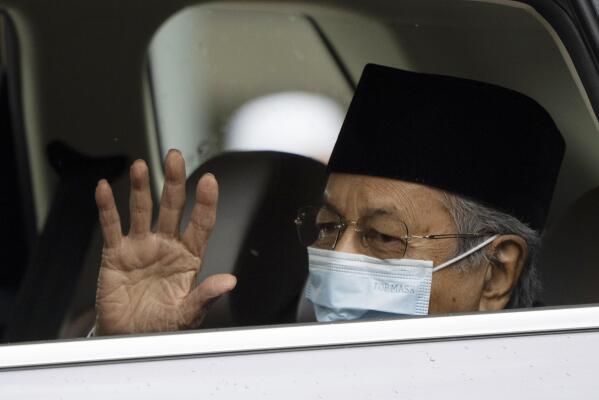The image features an elderly man with gray hair, wearing a rectangular-shaped black cap possibly for religious purposes, along with clear eyeglasses. His face is covered by a whitish-blue face mask, reminiscent of a COVID mask, which obscures his facial expression and makes it hard to determine his mood. He is seated in the backseat of a white vehicle, possibly a car, and the surrounding elements suggest he is near a window. To his left, his wrinkled hand is raised in a wave, as if greeting or bidding farewell to someone. The vehicle has black leather seats, one of which is visible and appears empty next to him. The background includes the framing and casing of the vehicle's door and window, adding to the confined atmosphere of the setting.